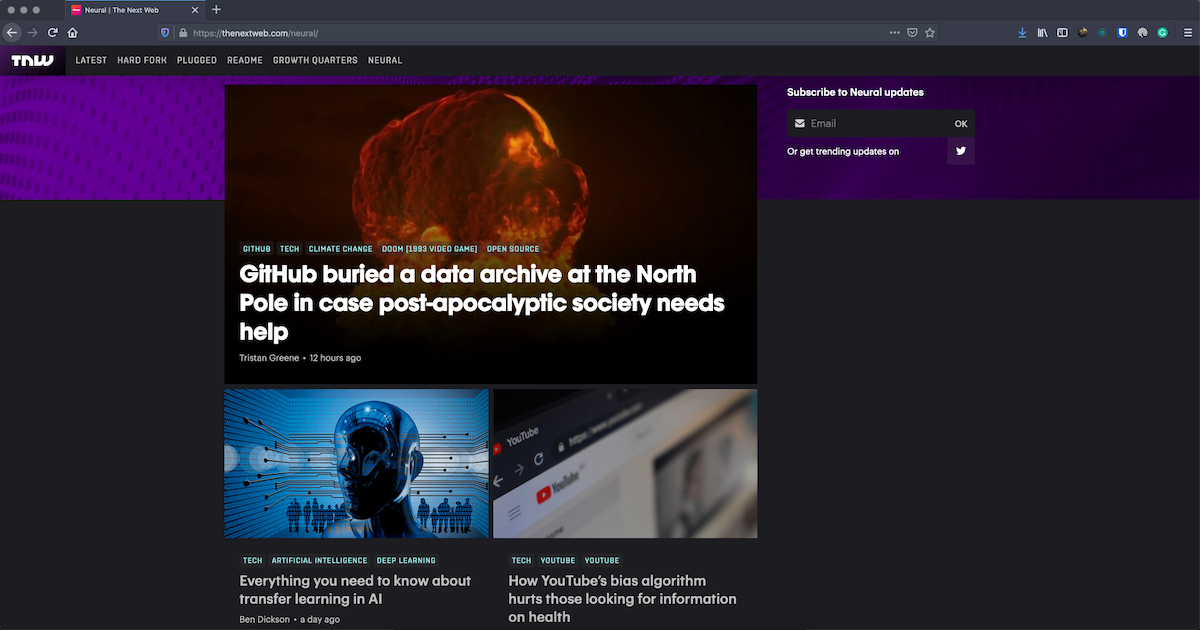This is an image of a rectangular website interface showcasing content from The Next Web (TNW) at the URL thenextweb.com/neural/. The header of the website features various categories listed from left to right: Our Latest, Hard Fork, Plugged, Readme, Growth Quarters, and Neural. The left side of the webpage starts with a black section, transitioning into the main content area in the center.

Prominently displayed is a headline image with the title, "GitHub Buried a Data Archive at the North Pole in Case Post-Apocalyptic Society Needs Help." Below this headline image, there are two smaller, split images. The layout and content focus on delivering a visually organized array of the latest articles and images under the Neural category.